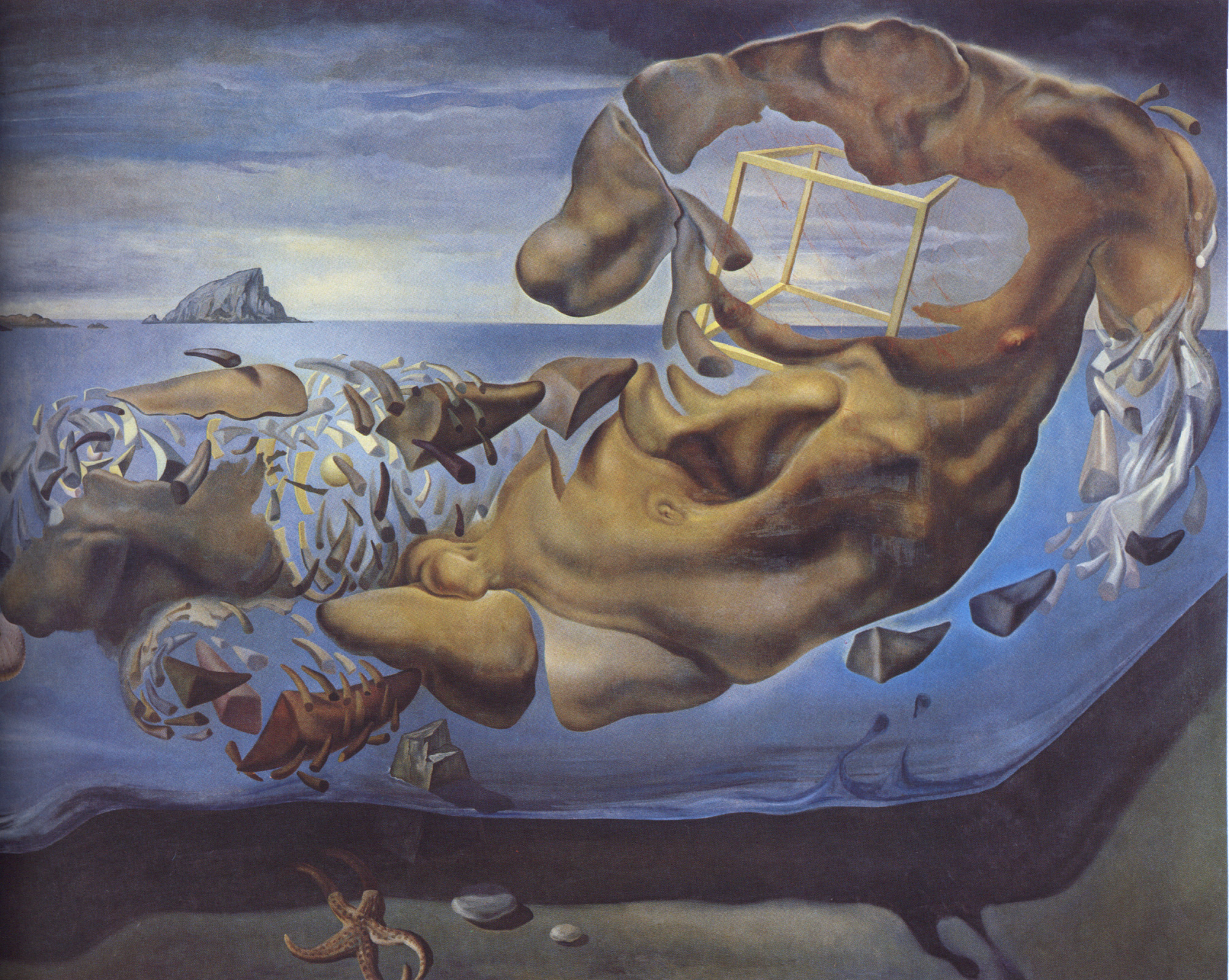The painting is an abstract and surreal depiction of a disintegrating nude male body set against a dark, cloudy sky. The figure, which appears to be made of clay, has its right leg, left arm, and portions of its chest and right arm disintegrating, revealing an empty chest cavity with a geometric square shape visible through it. The environment features an ocean scene at the bottom, with a dark shadow indicating the ocean floor, which is greenish-brown and contains an octopus, shells, and multiple bones of sea creatures. The water also includes a rock sticking out and a random large yellow cube outline. To the left, the distance reveals a rock structure, adding to the depth and complexity of the setting. The left arm of the disintegrating man appears to be composed of a swirling mass of metallic cylinders, and other body parts are scattered nearby, blending into the seabed. The entire scene channels an eerie, dream-like quality, merging elements of decay, nature, and geometric abstraction into a haunting tableau.